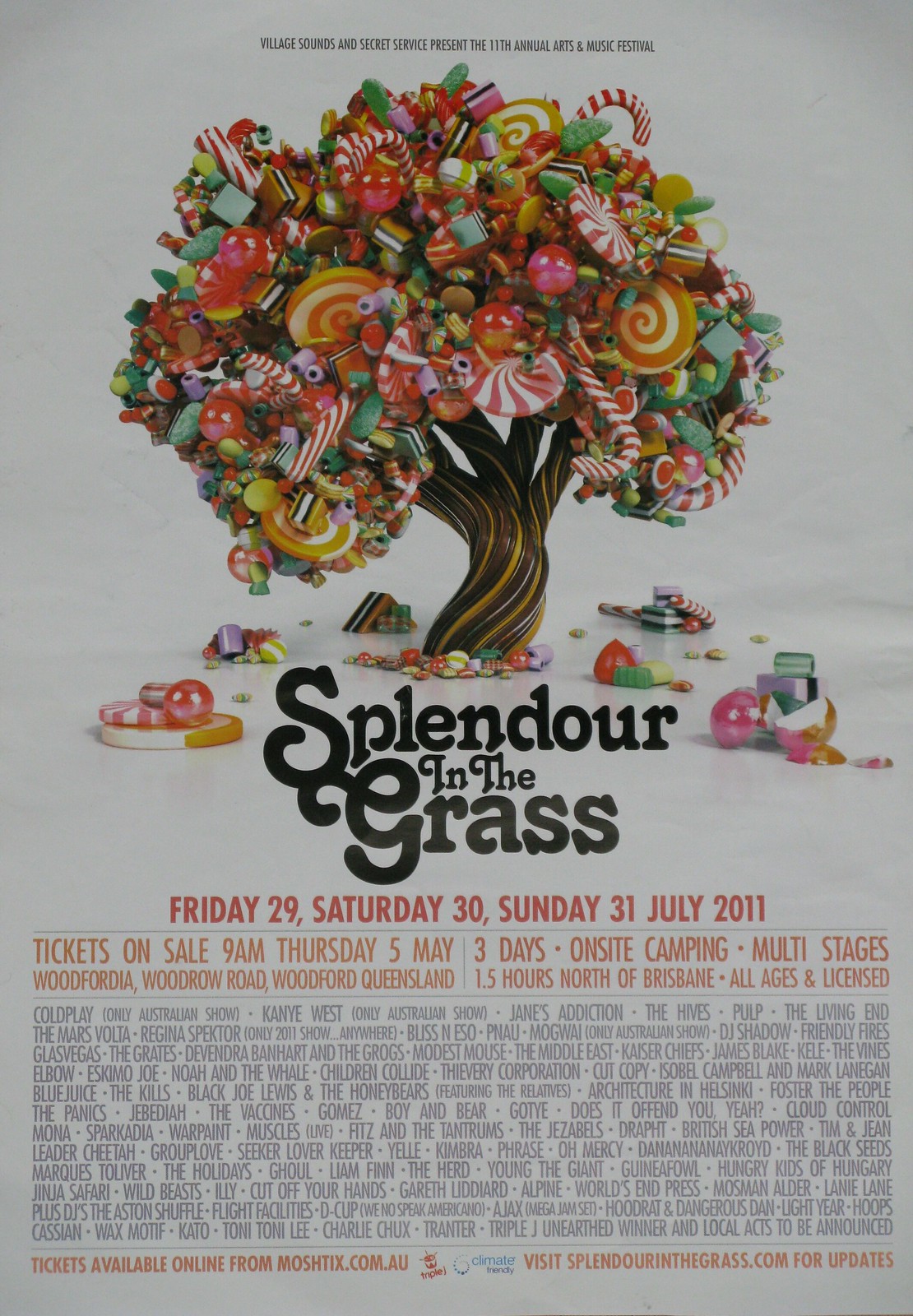The image is a scanned poster for the Village Sounds and Secret Service's 11th Annual Arts and Music Festival. At the top, there's small black text reading, "Village Sounds and Secret Service present the 11th Annual Arts and Music Festival." Below this text is a visually striking picture of a tree where instead of leaves, various candies are growing. The tree trunk appears to be crafted from brown, twisted material resembling Twizzlers or Red Vines, while the tree’s foliage consists of colorful candies, including lollipops, candy canes, bonbons, jelly candies, and gumballs in vibrant reds, greens, yellows, oranges, and whites. Candies are also depicted falling around the tree.

Beneath the tree image, bold black text announces "Splendor in the Grass," followed by red text listing the festival dates: "Friday 29th, Saturday 30th, Sunday 31st, July 2011." Below this, in orange text, it says, "Tickets go on sale 9 a.m. Thursday, 5th May." Further details note "three days on-site camping, multi-stages" at "Woodfordia, Woodrow Road, Woodford, Queensland," located "1.5 hours north of Brisbane." The event is described as "all ages and licensed," with additional information provided in fine print at the bottom, including website details.